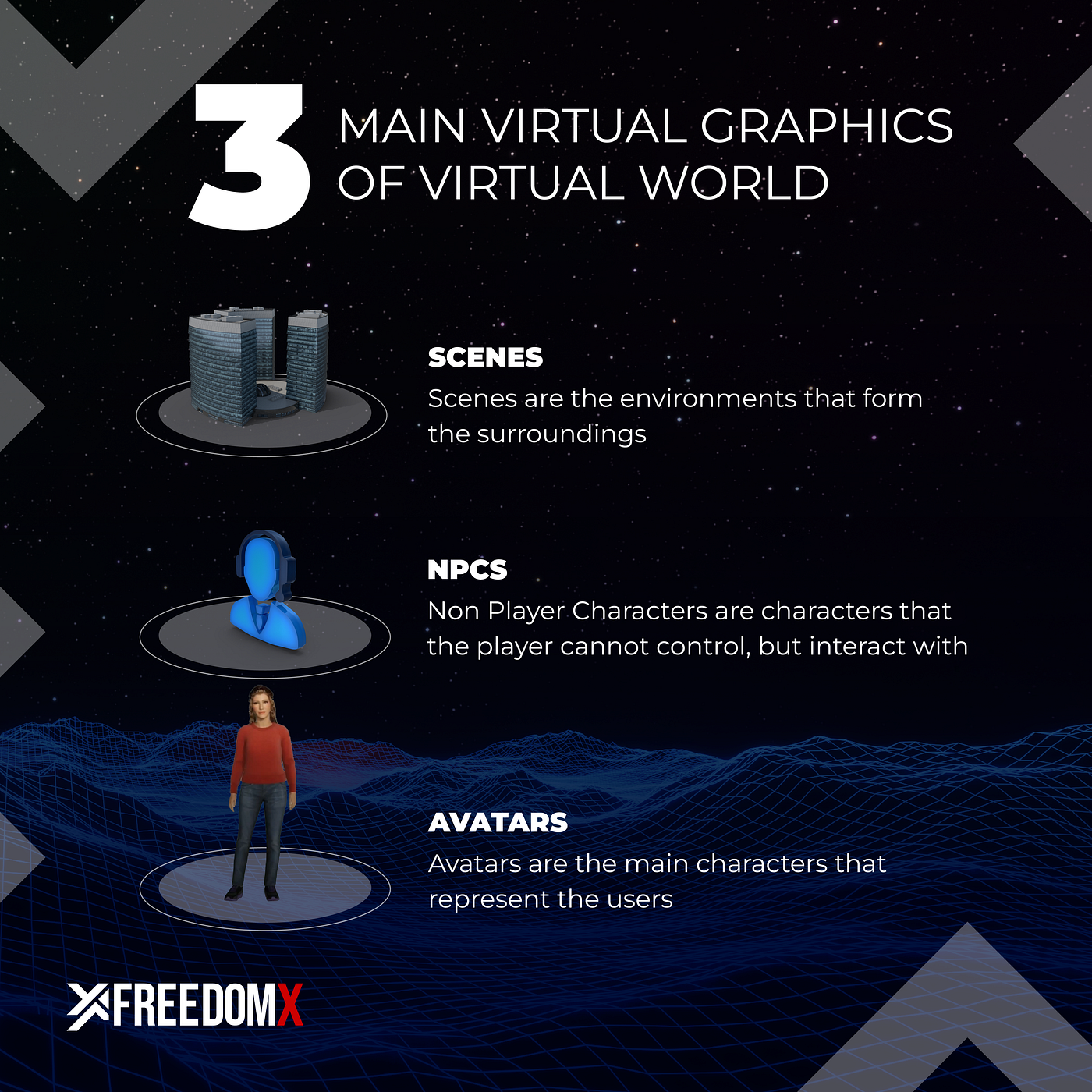The infographic, produced by Freedom X, is titled "Three Main Virtual Graphics of the Virtual World" and features a detailed, starry black background with silver dots and blue grid topography at the bottom. The infographic is divided into three main sections, each illustrating a different element of virtual graphics.

At the top, a title is followed by a graphic of three skyscraper buildings, labeled "Scenes." The description reads: "Scenes are the environments that form the surroundings."

The second section features an icon of a blue, faceless head and shoulders, representing "NPCs." The accompanying text explains: "Non-Player Characters are characters that the player cannot control but interact with."

The third graphic portrays a 3D-rendered woman with medium brown skin, wearing a red sweater and jeans, standing on a platform under the heading "Avatars." The text here states: "Avatars are the main characters that represent the users."

In the bottom left corner, the branding "Freedom X" is prominently displayed.